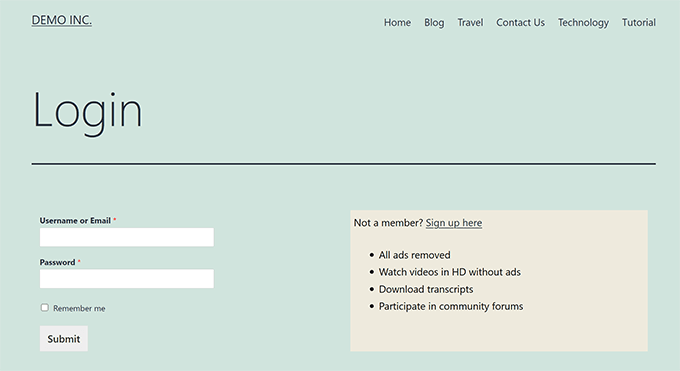The image portrays the login page for Demo Inc., featuring a clean, minimalist design. At the upper left-hand corner, the company name "DEMO INC." is prominently displayed in all capital letters with a black font, underscored by a thin black line. Adjacent to it, on the upper right-hand corner, is a horizontally justified menu bar containing links to Home, Blog, Travel, Contact Us, Technology, and Tutorial.

The background of the entire page is a light green, providing a fresh, inviting contrast. Directly under "DEMO INC." on the left-hand side is the word "LOGIN" in a large, thin font with a beginning capital 'L'. Following this is a small vertical space, then a thin black separator line, another small space, and the login form itself.

The left-aligned form starts with a text input box labeled "Username or Email." Below this is another input box labeled "Password" for password entry. Finally, at the lower left of the form is a gray "Submit" button, completing the clean and functional layout of the login page.